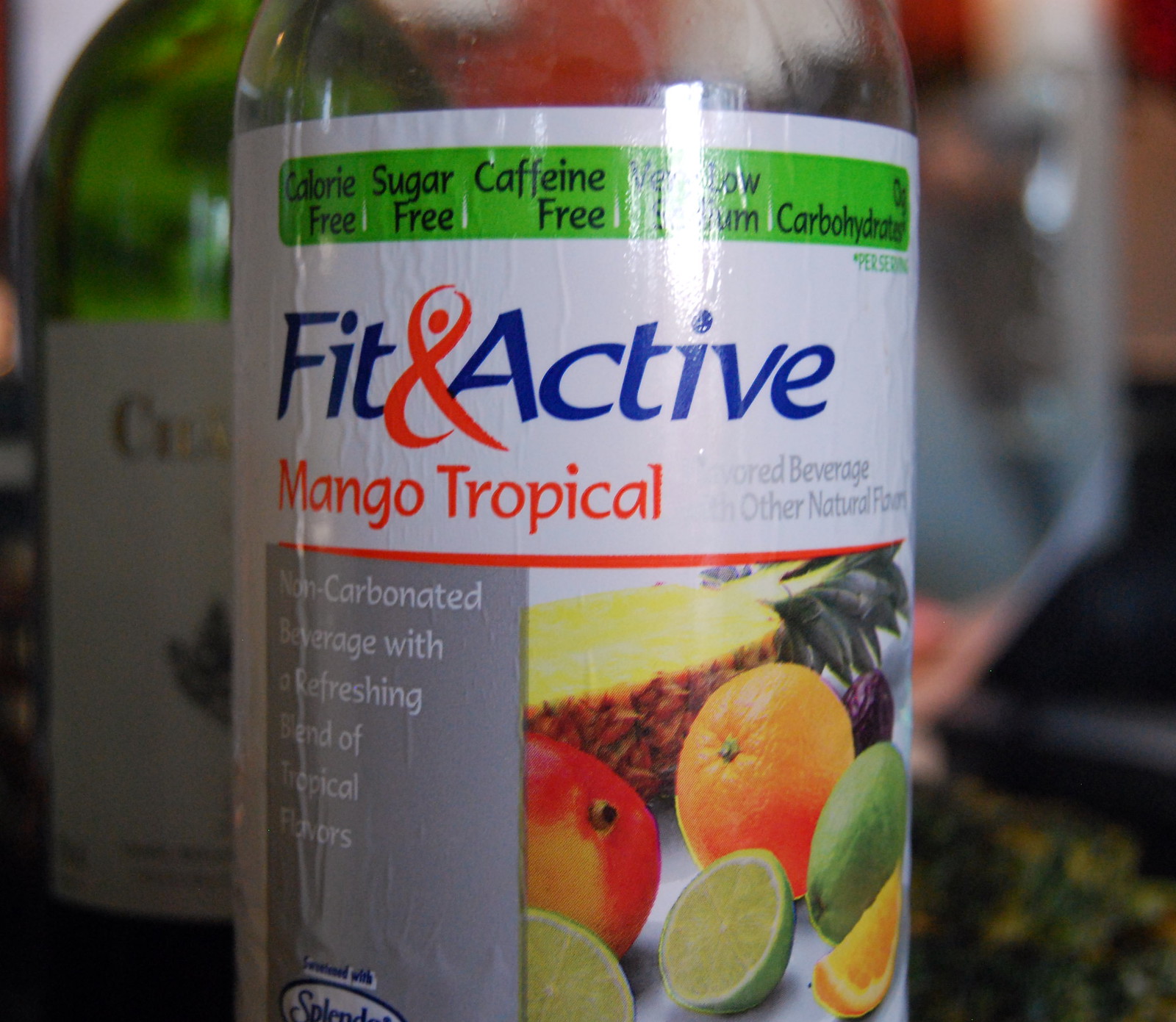The image features a close-up of a clear plastic bottle with a light green horizontal rectangular label. The label prominently displays black text indicating "calorie-free," "sugar-free," "caffeine-free," and "carbohydrates" on the right. Centralized on the label are the words "fit" in blue, followed by a red "@" symbol, and then "active" in blue. Directly below, the label reads "mango tropical" in bright red, with a small, faded gray text stating "flavored beverage, other natural flavors." A red line separates this segment from a vivid illustration of fruit, including an orange, a peach, lemons, limes, and a slice of pineapple. On the left, the label emphasizes the beverage as "non-carbohydrate" with a "refreshing blend of tropical flavors" against a gray background. In the background, to the right, another bottle with a green body and white label is partially visible, along with several indistinct green, black, gray, and red objects in the top right corner.